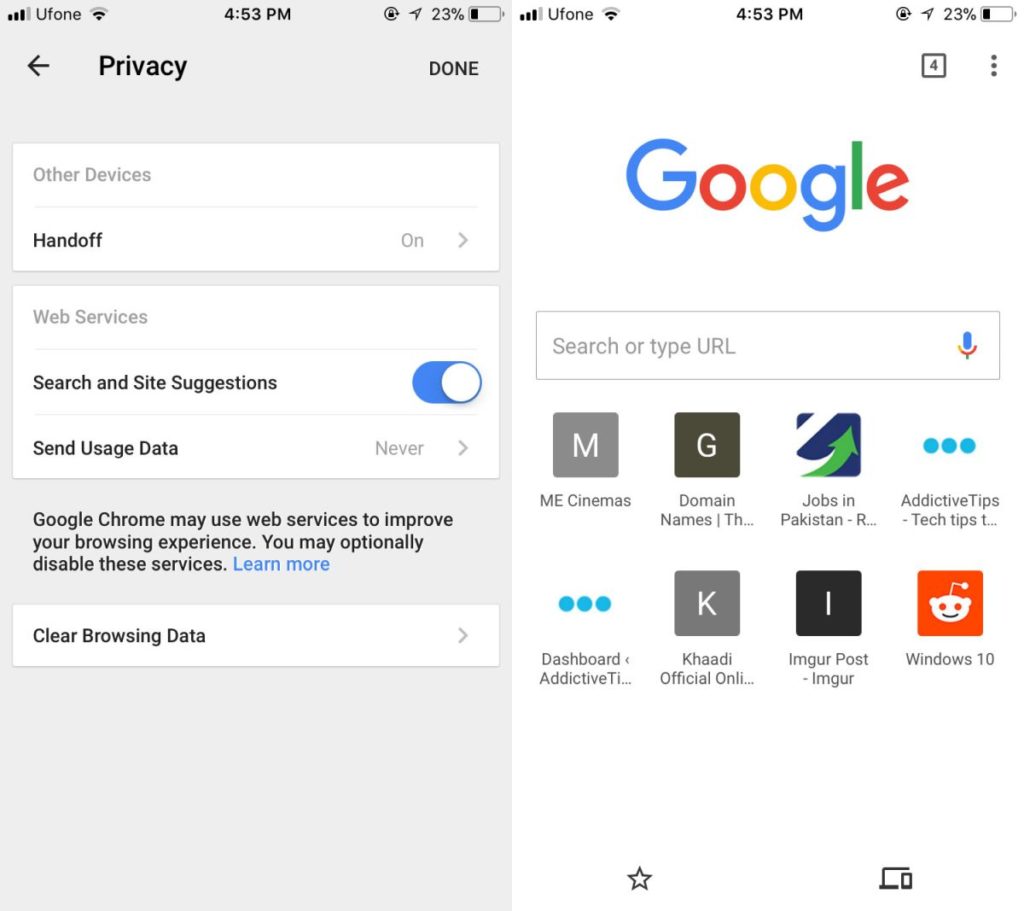This image is a composite screenshot taken from Google, divided into two distinct sections. The left section displays a user settings menu with a gray background. The menu features headings and options such as "Privacy," "Other Devices," and "Hand Off." It includes various toggles and settings: 

- A switch for "Web Services," which is turned on.
- A statement indicating that Google Chrome may utilize web services to enhance the browsing experience, with an option to disable these services and a "Learn more" link.
- An option to "Clear Browsing Data."
- A setting for "Send Usage Data" with the option "Never" selected.

The right section of the image shows the Google logo prominently displayed at the top, using its iconic blue, red, yellow, blue, green, and red letters. Below the logo is a search bar with a placeholder text, "Search or type URL." Beneath the search bar, there is a list of recent searches or bookmarks:

- ME Cinemas
- Domain Names
- Jobs in Pakistan
- Addictive Tips
- Tech Tips
- Dashboard
- Addictive Tips (repeated)
- Kadi Official Online
- Imgur Post
- Imgur
- Windows 10

The screenshot is entirely text-based, devoid of any photographic elements. There are no people, animals, birds, plants, flowers, trees, automobiles, or airplanes depicted in the image. Its primary focus is on the textual and interface elements related to Google Chrome settings and a typical Google search interface.